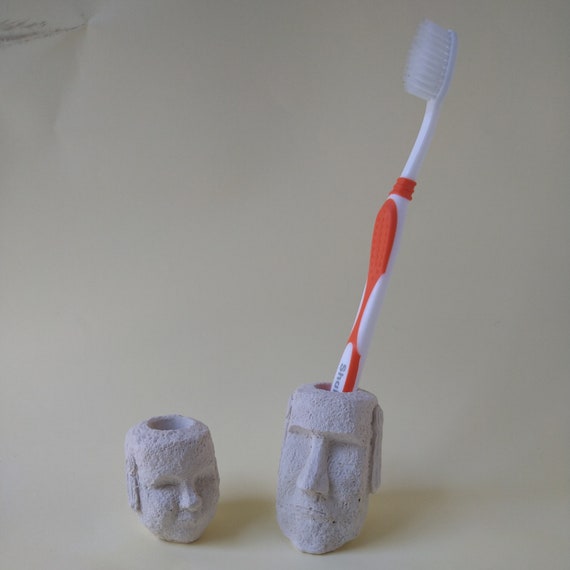This image captures a detailed scene featuring two rock-like toothbrush holders that resemble Easter Island statues. The smaller toothbrush holder on the left is empty, showcasing its hollow top. To its right stands a taller, similarly carved holder, also resembling an Easter Island head, containing a toothbrush. The toothbrush features a deep orange handle with white stripes transitioning into a fully white upper section, capped with clear, whitish bristles. These holders, sculpted from a pumice-type stone that gives them a light, nearly eggshell color, rest against a light beige-gray backdrop. The intricate stone faces present a contrast between the smaller, potentially feminine visage and the larger, more masculine one, adding an artistic flair to this domestic scene.